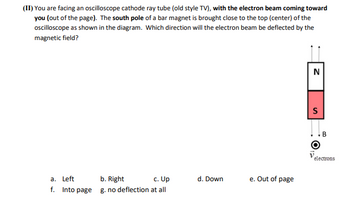The image features a multiple-choice question on a white background, resembling a test or quiz. On the right side, it includes a diagram with a horizontally split rectangle: the top half is white and labeled 'N' for North, and the bottom half is red or pink, labeled 'S' for South. The N section has two arrows pointing upward, while the S section has two arrows pointing downward. Additional labels indicate 'electrons' below the split rectangle. Gray dots are situated at the termini of the vertical lines extending from the ends of the N and S sections. 

The main text of the image reads: "You are facing an oscilloscope cathode ray tube (old-style TV) with the electron beam coming toward you out of the page. The south pole of a bar magnet is brought close to the top center of the oscilloscope, as shown in the diagram. Which direction will the electron beam be deflected by the magnetic field?" 

The provided answer choices are: 
A) Left 
B) Right 
C) Up 
D) Down 
E) Out of page 
F) Into page 
G) No deflection at all.